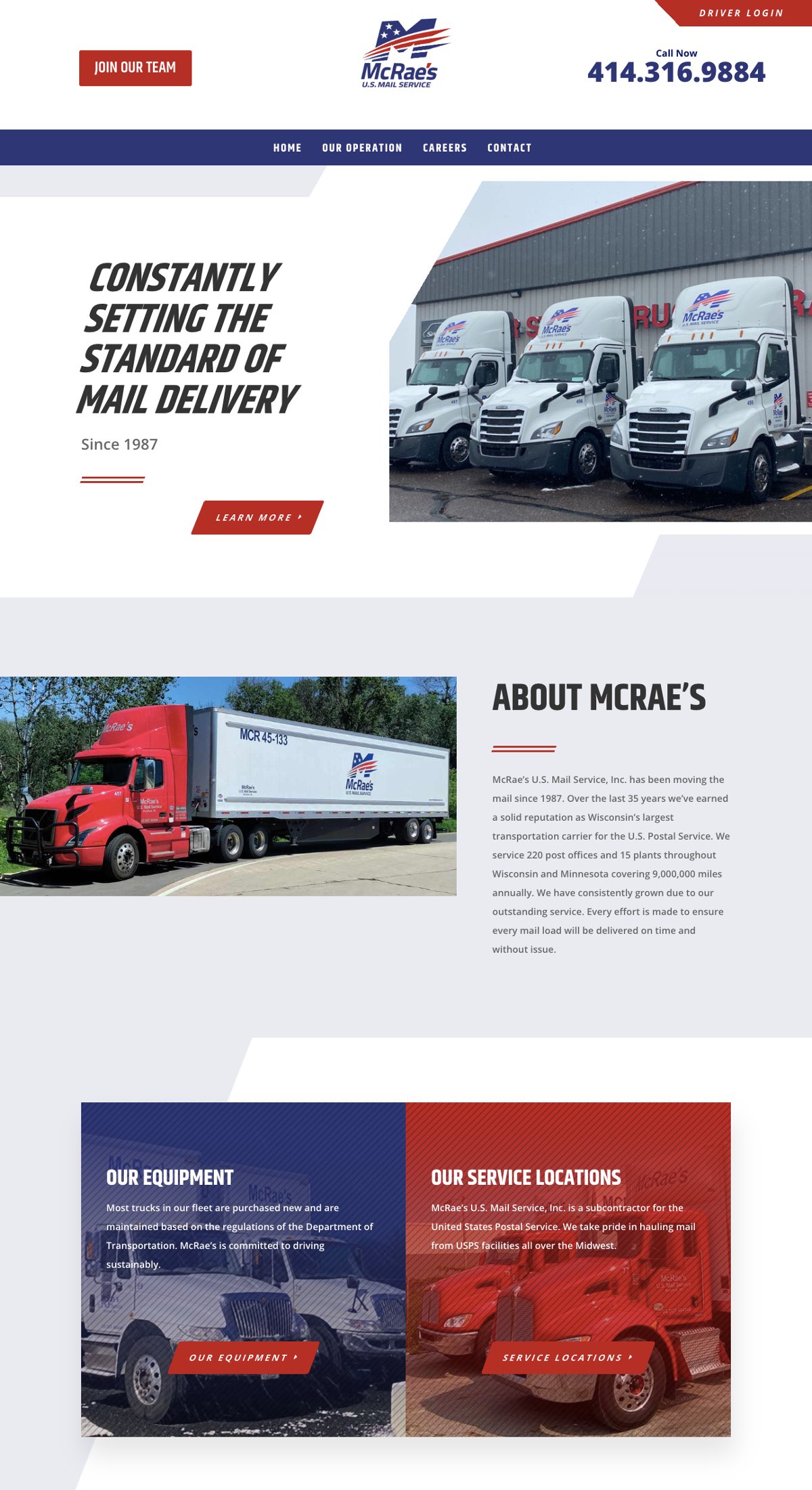The image showcases the website of Macraes, a prominent trucking company known for setting high standards in mail delivery and parcel transportation. Dominating the visual space are multiple photographs of semi-trucks, some hitched to trailers and others unhitched, either parked in a lot or on the open road. The fleet primarily consists of white trucks, although there are notable appearances of red trucks as well, contributing to a bold color palette interspersed with red, white, and blue—a nod to a patriotic theme present in the company's branding.

The Macraes logo is prominently featured, incorporating a stylized 'M' with stars and diagonal red stripes against a blue backdrop, reinforcing the company's American ethos. Key navigational elements include a 'Driver Login' button positioned at the top right, a conspicuous red 'Join Our Team' button on the top left, and a visible phone number for direct contact.

The website appears to be divided into main sections such as "About Macraes," "Our Equipment," and "Service Locations," each offering links for more extensive information. Though much of the finer text remains unreadable, the emphasis on mail delivery and potentially large package transportation is clear.